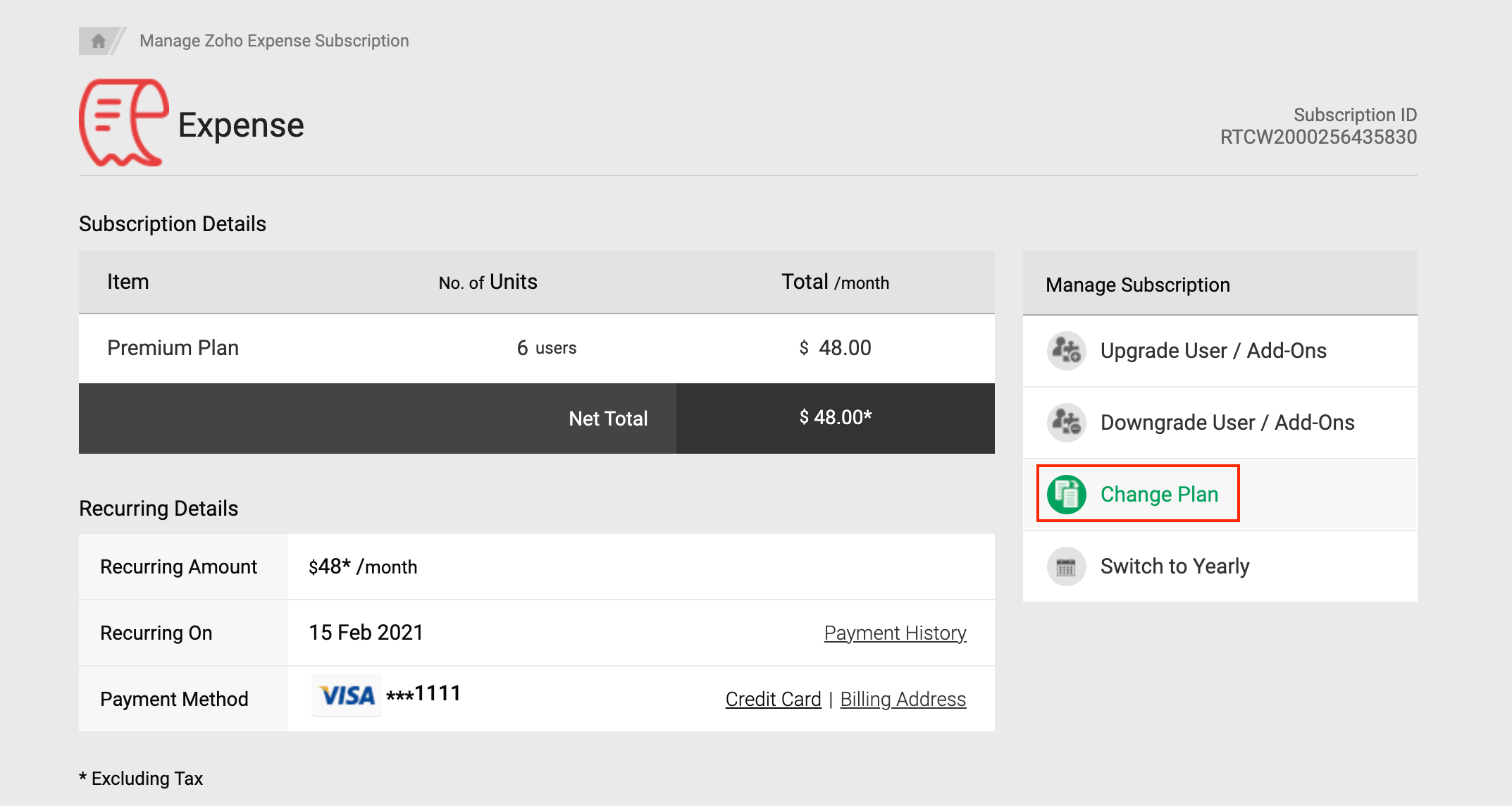Screenshot of a confirmation page detailing a subscription plan for Zoho Expense. The heading at the top left reads "Manage ZOHO Expense Subscription," while the top right displays a unique subscription ID number. Below the heading, the subscription details are outlined.

The item being purchased is identified as a "Premium Plan" for six users, with a total cost of $48 per month. Consequently, the net total amounts to $48 monthly. 

Further down, there's a section for recurring payment details. Here, it is specified that the amount of $48 will be charged monthly, recurring on the 15th of each month starting from February 15th, 2021. 

Additional links and details are available for payment history. The payment method specified is a Visa card ending in 1111. On the right side of the page, various management options are provided, including "Upgrade User Add-ons," "Downgrade User Add-ons," "Change Plan," and "Switch to Yearly."

Note: The mentioned amount does not include tax.